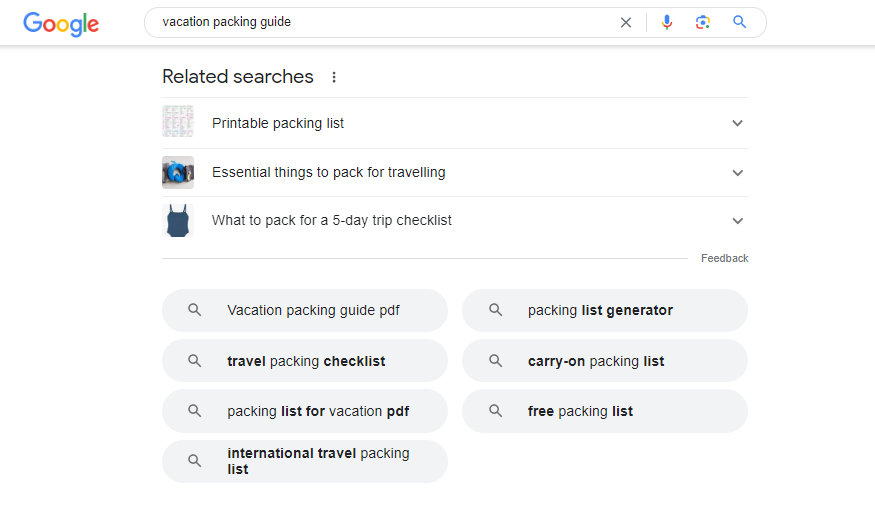The image depicts a Google search results page for the query "vacation packing guide." At the top left corner of the screen, the familiar "Google" logo is visible. In the search bar, the text "vacation packing guide" is entered, with an 'X' icon to clear the search, a microphone icon for voice input, an unspecified symbol (possibly a camera for image search), and a magnifying glass icon for initiating the search.

Below the search bar, the section titled "Related searches" includes several suggested search queries. The first suggestion is "printable packing list," followed by "essential things to pack for traveling," and "what to pack for a five-day trip checklist."

Further down, there are seven horizontally aligned ovals, each accompanied by a small magnifying glass icon, indicating clickable search options. These ovals contain the following search phrases from left to right:
1. "vacation packing guide PDF"
2. "travel packing checklist"
3. "packing list vacation PDF"
4. "international travel packing list"
5. "packing list generator"
6. "carry on packing list"
7. "free packing list"